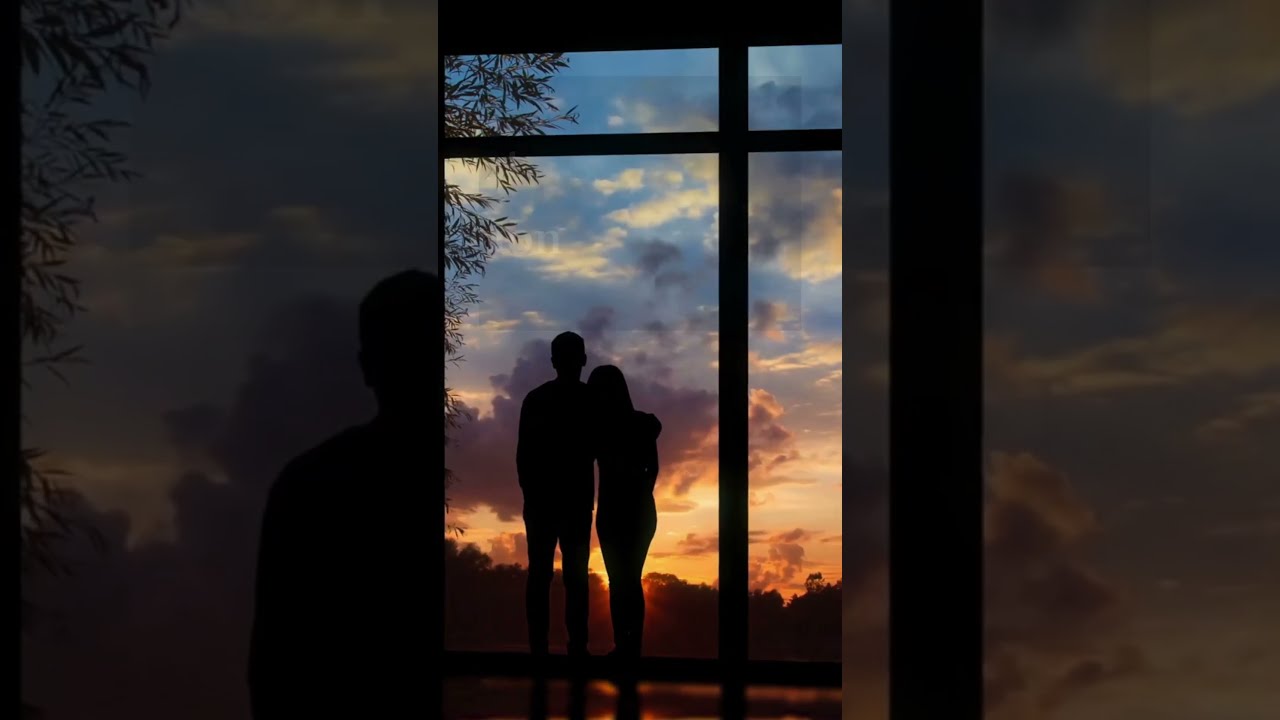In this evocative photograph, a couple stands side by side, backlit by a breathtaking sunset through a large floor-to-ceiling window. The man, taller and on the left, lovingly wraps his right arm around the shorter woman on the right, who gently leans her head on his shoulder. Their forms are rendered as black silhouettes, obscuring any specific details about their faces or clothing, leaving only their intimate posture visible. The sky outside transitions smoothly from a soft light blue at the top to vibrant pink and orange hues near the horizon. A brilliant yellow-orange sun sets just above a distant tree line, casting a warm glow. The scene is framed elegantly by a border that consists of zoomed-in and slightly grayed-out elements of the central sunset image, adding depth and focus to the heartfelt moment they share. Branches from a nearby tree intrude slightly into the upper left corner, emphasizing the natural beauty surrounding them.